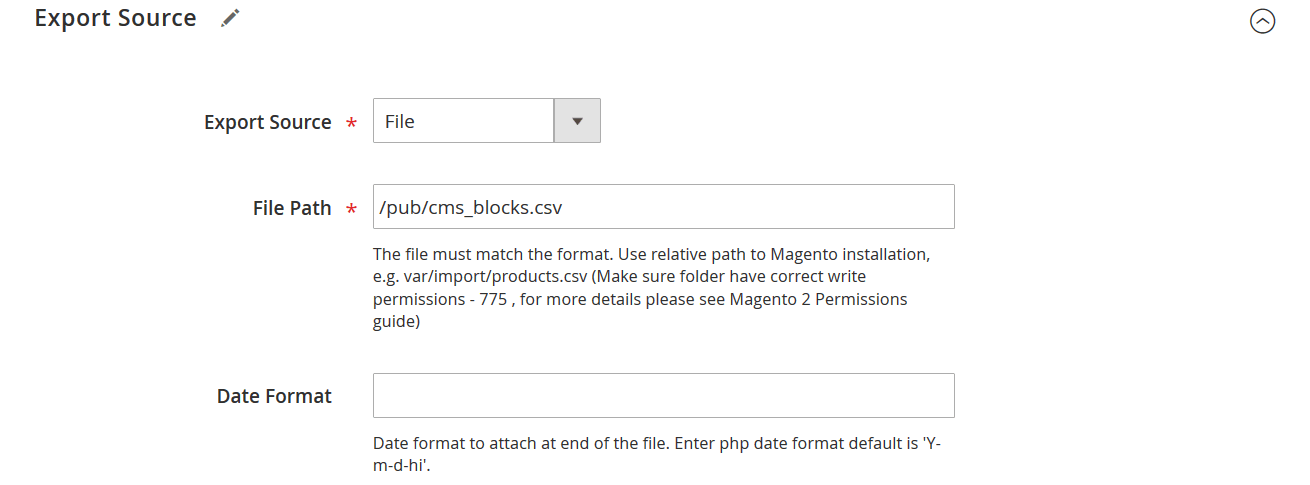The image is a horizontally rectangular screenshot of an export window with a white background. At the top left corner, the text "Export Source" is displayed in black, accompanied by an edit icon. Directly across on the far right, there is an upload icon (an upward-pointing arrow encircled by a circle). Below this header, the main section of the window includes the "Export Source" label with a corresponding input field to its right, featuring a dropdown option for file selection.

Next to the "Export Source" label and its input field, there's a "File Path" label accompanied by another input field. Instructions beneath this specify that the file must match the specific format and advise users to use a relative path to the Magento installation. Both "Export Source" and "File Path" labels are marked with red asterisks, indicating that these fields are mandatory.

Towards the bottom of the window, there is a "Date Format" label followed by an input field designated for the date format. Instructions just below this field indicate that the date format entered will be attached to the end of the file and should be entered in PHP date format. The default date format is given as "Y-M-D-H-I".